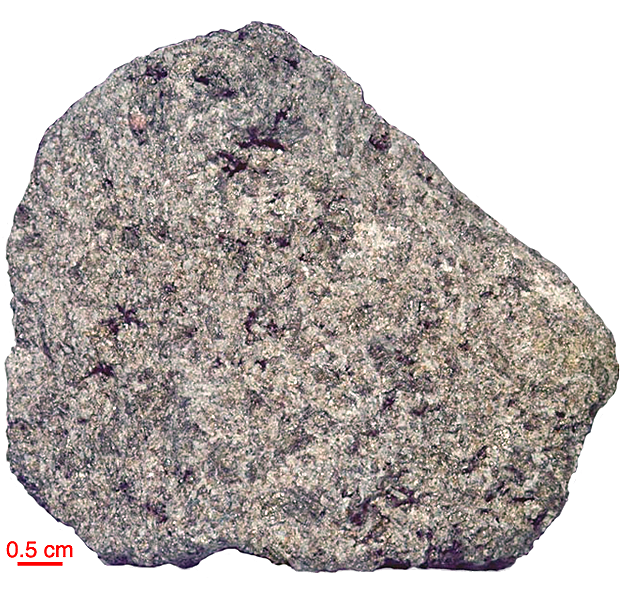The image features a singular rock presented against a pure white background, reminiscent of a textbook or stock photo. The rock, which predominantly displays shades of gray, is embedded with small white and gold flecks. Sparse red markings are subtly visible, the rarest of the colors present. Its shape is somewhat rounded but not a perfect circle, with a jagged and rough texture indicating a hard material. The rock also exhibits touches of black, green, muted yellow, and brown, contributing to its diverse appearance. In the bottom left corner of the image, the rock's size is indicated in bright red text, reading "0.5 cm" with a red line underscoring the measurement.